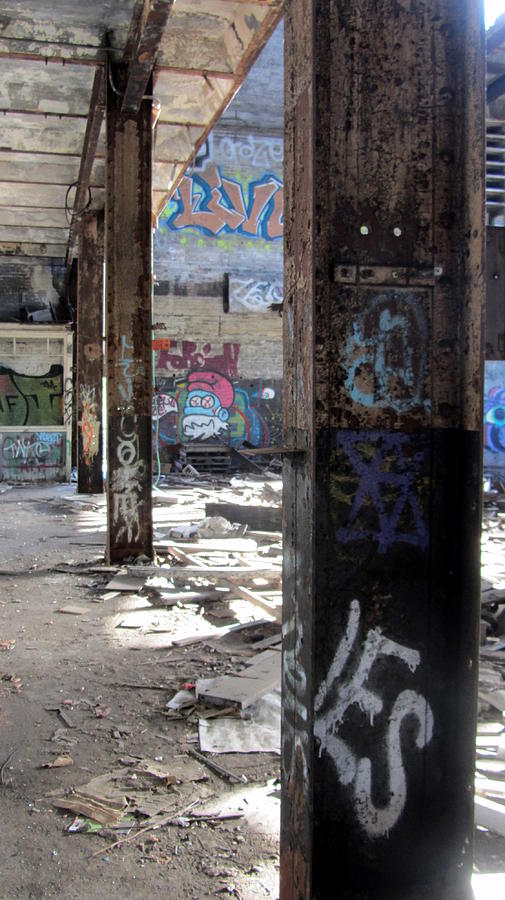The photograph captures a grungy, abandoned urban setting, likely either a warehouse or the underside of a bridge, characterized by its high, black steel support columns covered in graffiti. These columns, possibly metal, are arranged in a receding line that enhances the depth of the image, with three prominently visible. The floor, made of gray cement or stone, is littered with newspapers, trash, and dirt, emphasizing the neglected state of the area. In the background, a tan brick wall, also covered in graffiti, features distinctive artwork, including a depiction of a smurf-like blue person with a white beard and a red hat at the bottom, and an orange, lettered tag that appears to spell "life" higher up. The ceiling above these columns transitions from white to sections covered in blue and orange graffiti, adding to the chaotic urban aesthetic.